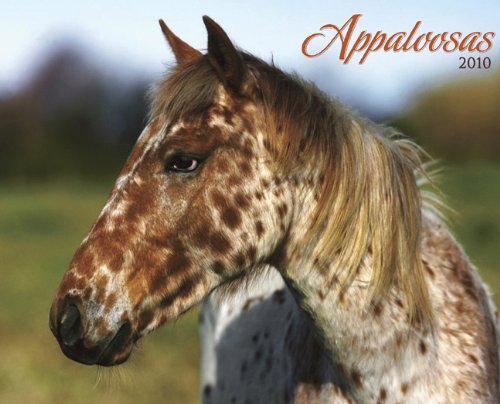This photograph, likely designed for an advertisement or calendar cover, features a striking Appaloosa horse with distinct coloring and notable text in the upper right corner that reads "Appaloosa's 2010" in red and black lettering. The horse dominates the image, positioned in a green pasture with trees in the background, indicative of a spring or summertime setting. Its head, slightly turned to the left, reveals a close-up of its expressive face, which is mostly brown with contrasting white spots. The mane is a mix of light brown and blonde streaks. The rest of the horse's body, extending into the shot, is primarily white adorned with brown spots, particularly along its neck and back, although there is some brown along its back. The detailed pattern on its coat and the natural outdoor scenery combine to give the impression of an idyllic farm setting, further enhanced by the lush green grass and distant trees.